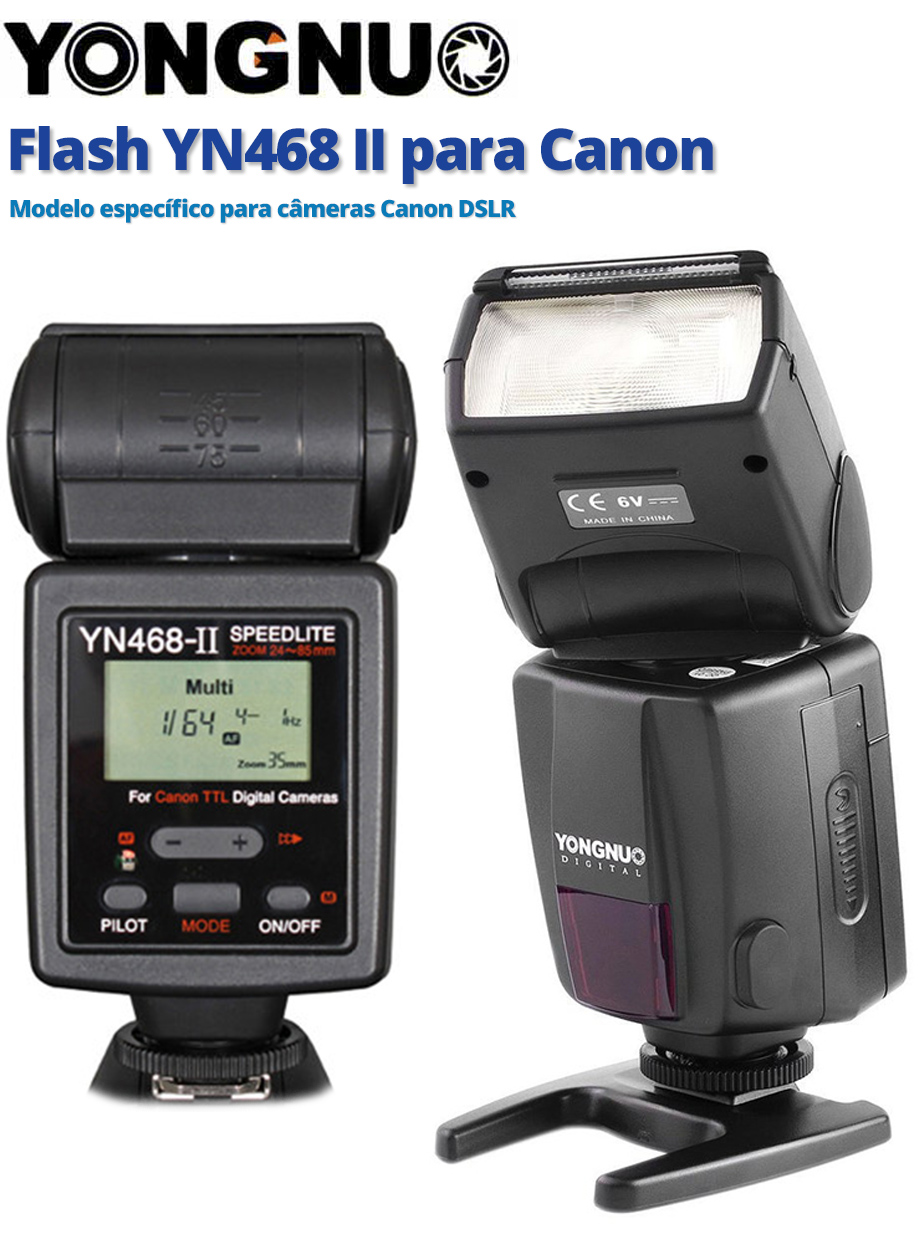This is a detailed photographic advertisement for a Yongnuo YN468 II Speedlight, specifically designed for Canon DSLR cameras. The prominent branding, Yongnuo, spelled Y-O-N-G-N-U with an iris symbol at the end, is displayed across the ad. The flash unit, model YN468 II, is accompanied by the text "Modelo Especifico Para Cameras Canon DSLR," emphasizing its compatibility with Canon digital single-lens reflex cameras.

The image showcases both the front and back of the flash unit, highlighting various features and controls. The back of the unit features a digital display screen with "Multi 64," and control buttons labeled Pilot, Mode, and On/Off for easy operation with Canon TTL digital cameras. The flash unit can pivot to enable a bounce effect, enhancing lighting flexibility.

The flash’s design is described in detail: it has a square shape with a mounted black plastic piece supporting it, featuring adjustable knobs that allow for a 360-degree swivel. The unit also includes a zoom feature and an adjustable top part for angling the flash upwards or downwards. The stand at the base permits stable placement, enabling remote setup when necessary.

The front of the flash unit includes a red sensor and is predominantly black with a sleek plastic finish. The combination of the practical stand, swivel button on the head, and controls make this Speedlight a versatile tool tailored for Canon DSLR users looking for precise and adaptable lighting solutions.